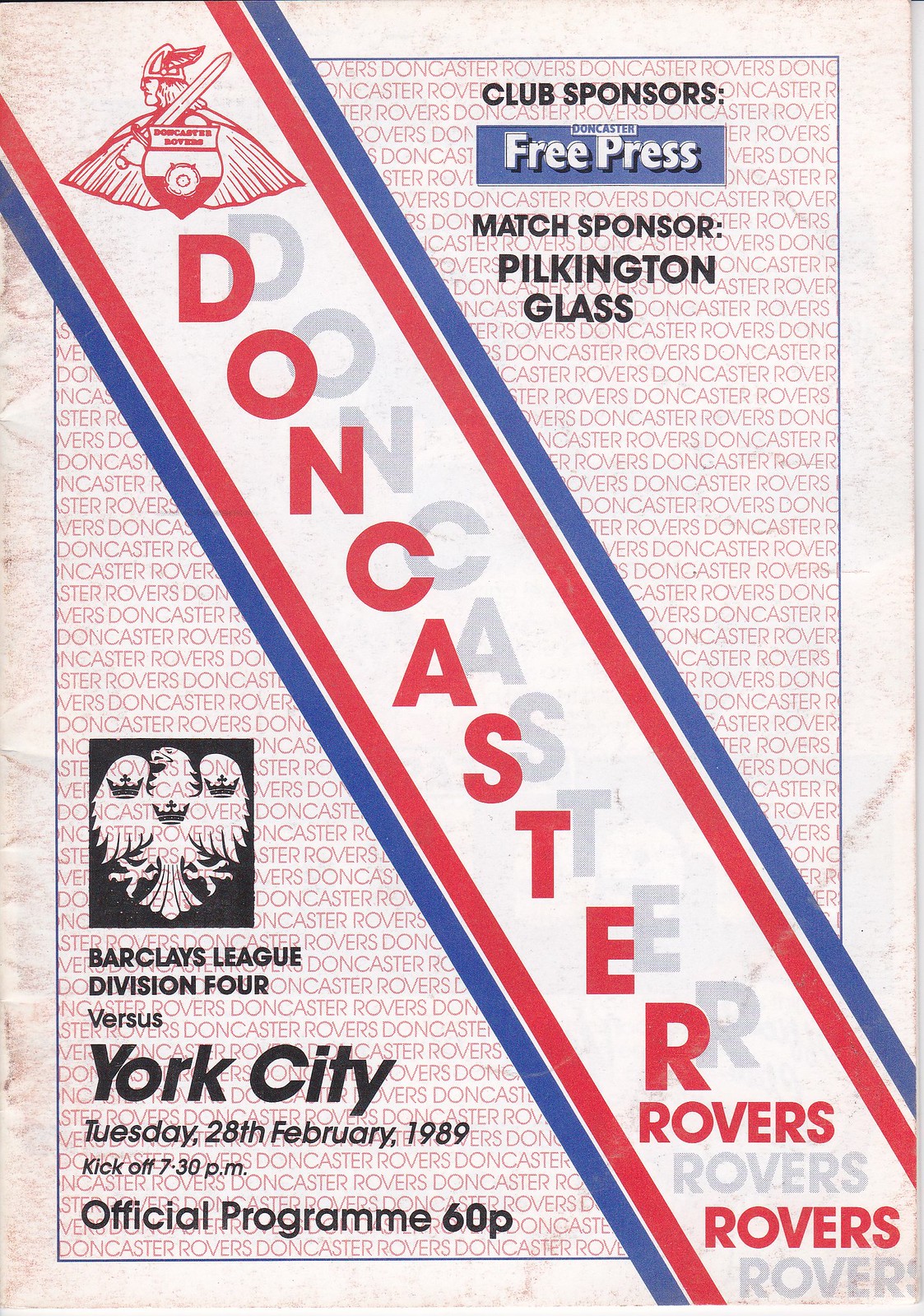This is an image of an official soccer program for a match between Doncaster Rovers and York City, scheduled for Tuesday, 28th February 1989, with kickoff at 7:30 p.m. The cover features a light background with "Doncaster Rovers" repeatedly inscribed in a faint font. A prominent diagonal banner extends from the upper left corner to the lower right corner, featuring red and blue borders and a white center with the name "Doncaster Rovers" written twice: once in light gray and once in bold red. Atop the banner, there's an illustration of a Viking. The upper right corner of the cover highlights the club sponsor, "Free Press," and below it, the match sponsor "Pilkington Glass" in black font. The lower left corner displays an eagle emblem along with the text "Barclays League Division 4 vs. York City," the match details, and "Official Program 60p."